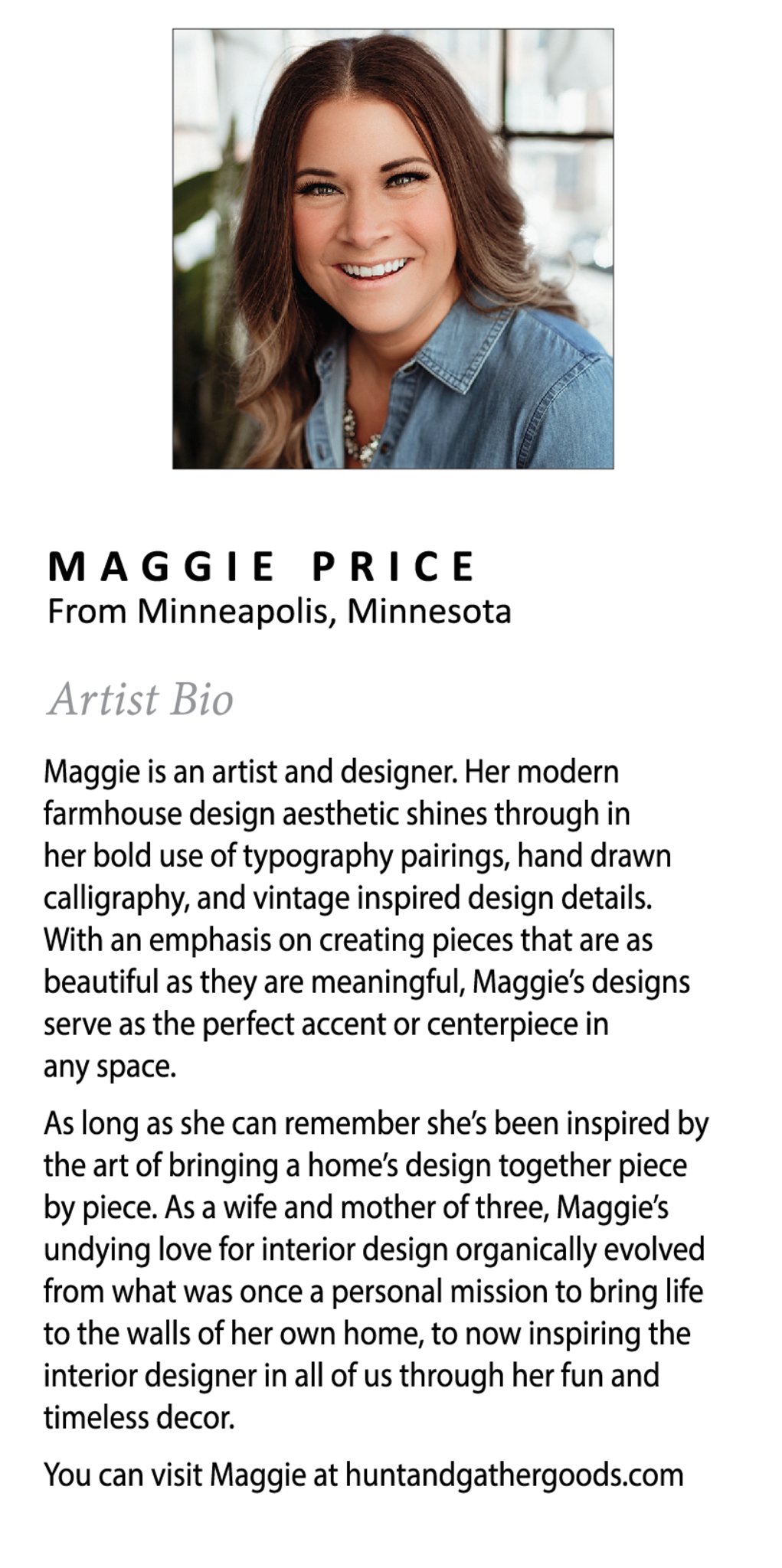The image displays a bio page featuring a headshot of a woman named Maggie Price from Minneapolis, Minnesota. She has long brown hair, light to medium skin tone, and is smiling with her teeth visible. Maggie is dressed in a blue, denim-style shirt with a collar. The background of the photo is entirely white, with a green room-type plant partially visible in the frame. Beneath her image, bold all-caps text reads "Maggie Price," followed by clear lettering indicating "From Minneapolis, Minnesota," and then "Artist Bio" in a light gray font. The accompanying bio details Maggie as an artist and designer known for her modern farmhouse aesthetic, characterized by bold use of typography, hand-drawn calligraphy, and vintage-inspired design elements. Her work emphasizes creating pieces that are both beautiful and meaningful, making perfect accents or centerpieces in any space. Additionally, the bio notes that as a wife and mother of three, Maggie's passion for interior design evolved from her personal mission to enliven her own home to inspiring others through her timeless decor. Additional paragraphs continue to elaborate on her artistic journey and provide a website for more information: huntandgathergoods.com.